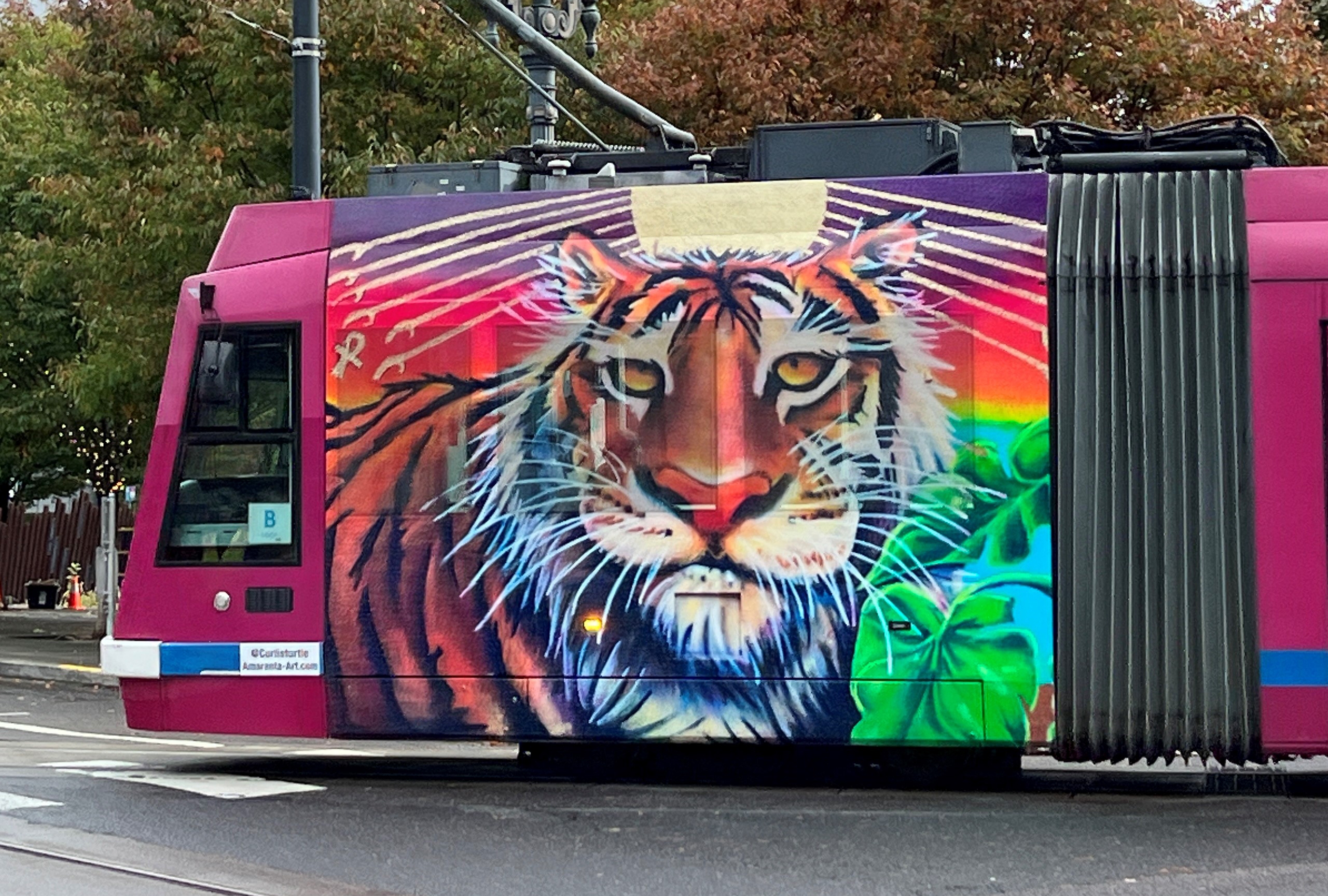The image captures a vibrant, outdoor scene dominated by a whimsically painted pink vehicle, likely a bus or a cable car, adorned with a detailed tiger graphic. The tiger boasts green eyes, prominent whiskers, and an expressive mouth, surrounded by artistic rays of the sun and lush green plants. The vehicle, notable for its pink hue and distinctive accordion-like midsection, lacks visible tires and features a uniquely shaped rectangular front window. A blue and white bar with unreadable text spans its side. In the background, trees transitioning to fall colors of green, brown, and reddish hues, frame the scene, with a street running below. The combination of real foliage and the bus's vibrant decor creates an eclectic and striking visual.